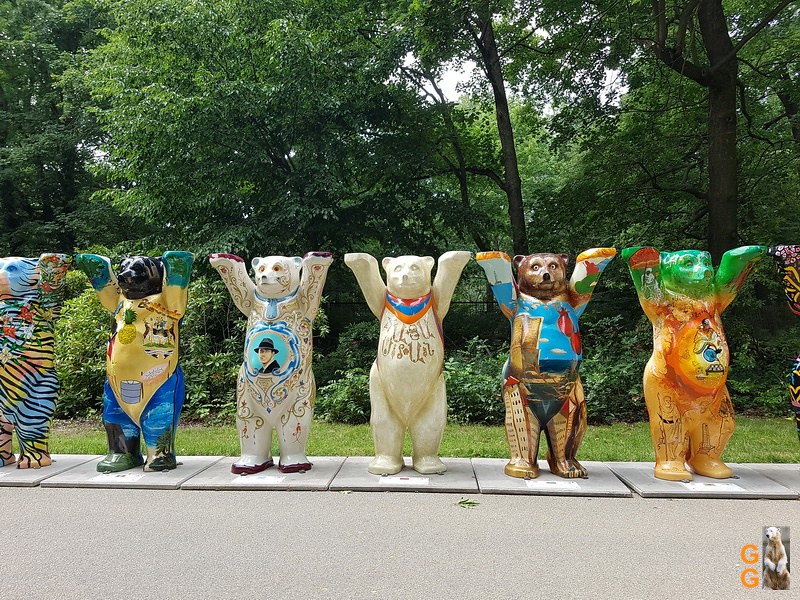This captivating outdoor photograph features a line of six creatively decorated bear statues, each uniquely painted and perched atop individual gray concrete blocks. The backdrop is a lush wooded area with dense clusters of trees, leafy green bushes, and a small grassy patch leading up to the platform where the bears stand. The statues are displayed on a white platform that rests on a gray pavement.

On the far left, the first bear, slightly cut off, is adorned with black stripes and vibrant hues of blue, yellow, and pink, decorated with floral designs. Next, the second bear showcases a tropical theme with a yellow belly featuring a pineapple, a black head, teal green hands, and blue legs. The third bear stands out with an all-white body decorated with floral patterns and a portrait of a man wearing a hat painted on its belly.

The fourth bear sports a clean, off-white look with a striking red, blue, and orange scarf painted around its neck. Moving on, the fifth bear has a brown head, a multicolored torso that includes shades of blue, red, and brown, and legs with intricate designs. Lastly, the bear on the right flaunts a neon green head, a yellow-orange base, and detailed graphics on its torso, including letters "GG" in orange on the bottom right, as well as some male figures.

All the bears are standing upright with their arms raised high toward their heads, creating a whimsical and visually engaging display.